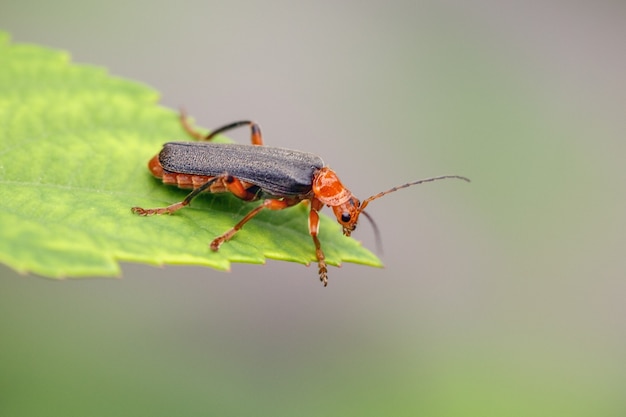This close-up photograph captures a striking beetle perched on the serrated tip of a bright green leaf that extends from the upper left side of the image. The beetle, predominantly in orange with a red-tinted body, boasts six orange legs and intricate red and black striped antennae sprouting from its head. Its black wings rest upon its back while its dark eyes, one clearly visible in the shot, gaze downward at the leaf's tip. The beetle's legs are detailed with fine hairs, adding texture to its appearance. The leaf itself displays slightly darker green veins against its bright surface. The background is an indistinct blend of gray, green, and muted purples, ensuring that the beetle and leaf are sharply in focus and the undeniable focal points of the image.